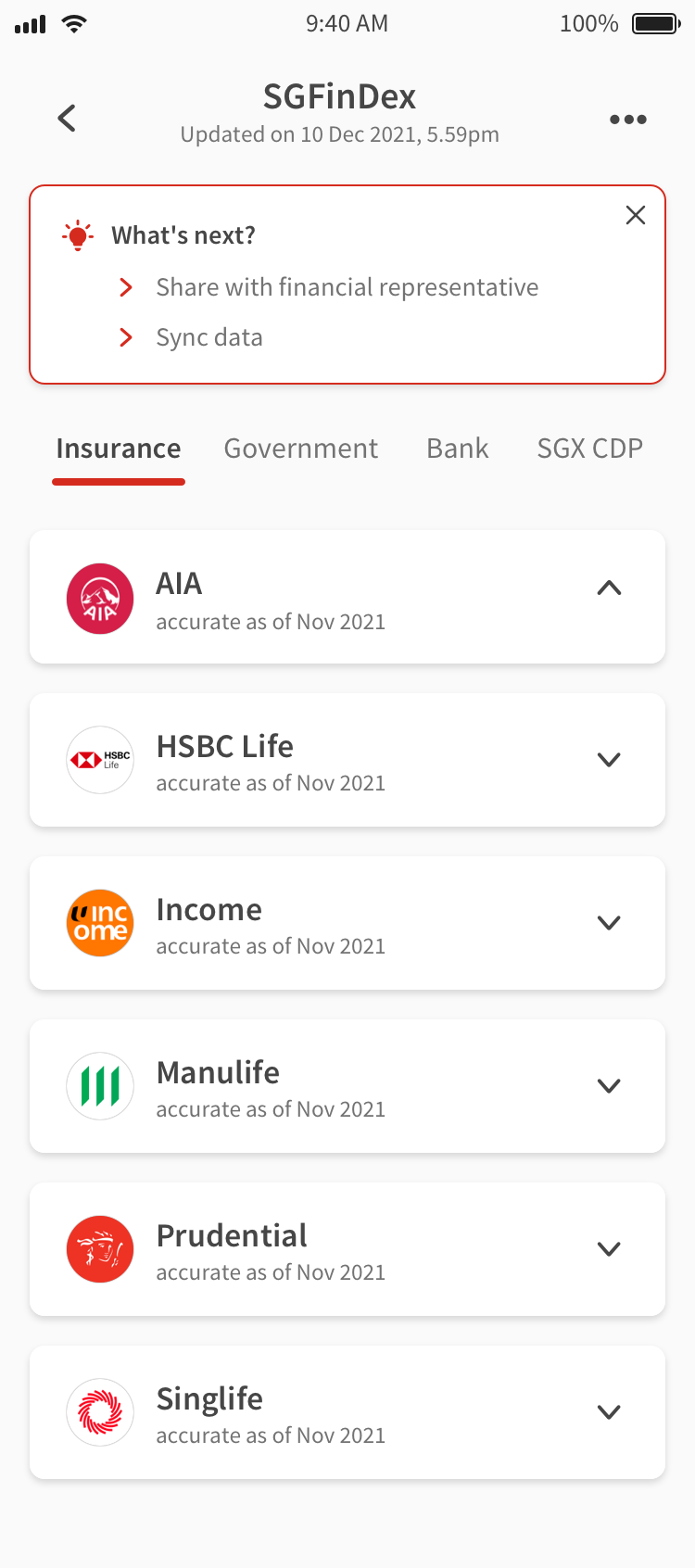The image displays a screenshot from an Apple mobile device showcasing a financial application interface. The status bar at the top indicates the phone has full cellular signal, full Wi-Fi signal, and a 100% battery level, with the time displayed as 9:40 AM.

Directly below the status bar is a navigation arrow pointing to the left, and to its right, it reads “Sgfindex”. It notes that the information was updated on December 10th, 2021, at 5:59 PM. To the right of this, there is an icon with three dots indicating more options.

The main highlighted feature on the page is marked in red and displays a red light bulb icon with the label "What Next?” accompanied by two small right arrows, also in red. The options "Share with financial representative" and "Sync data" are listed underneath.

Further down, a menu appears with the "Insurance" tab highlighted, next to other tabs labeled "Government", "Bank", "SGX CPD", each representing different sectors. The insurance section lists various financial companies:

1. **AIA** - Represented with a red circle, the icon displays the letters "AIA". Next to it is a label indicating "Accurate as of November 2021" with an arrow pointing up.

2. **HSBC Life** - Depicted with a red stop sign icon featuring a white hourglass lying on its side.

3. **Income** - Shown with an orange circle containing the word "Income" in white.

4. **Manulife** - Presented with a white circle containing green lines.

5. **Prudential** - Illustrated with a red circle showcasing a sketch of a lady.

6. **Singlife** - Exhibited with a red wreath on a white circle.

Except for AIA, the remaining listed companies have arrows pointing down, possibly indicating a downward trend or status update.

In summary, this screenshot is an interface from a financial application, intended for users to track and manage their insurance and other financial accounts across different institutions.